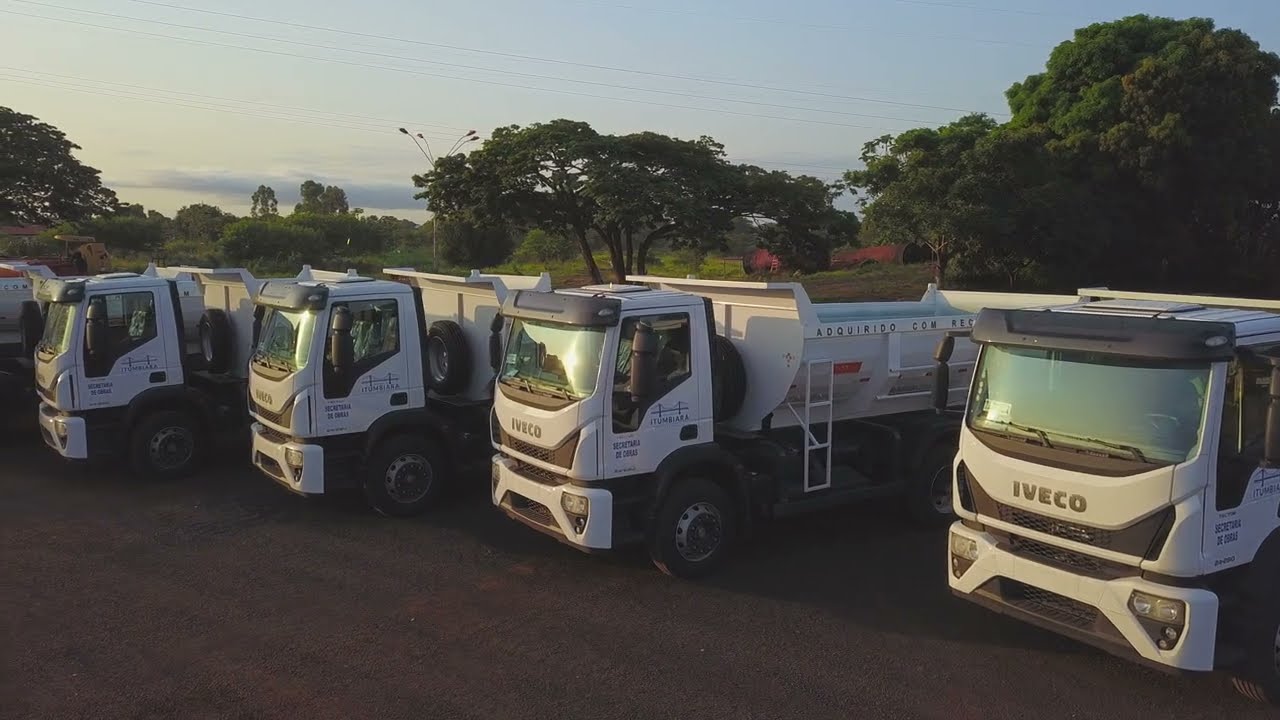The image captures a slightly elevated exterior shot, potentially from a second-floor building, providing a high-angle view of five Iveco dump trucks parked diagonally in a row. Each truck features a flat front with white bodies and black trims, including a black grill and wind visor. The trucks have large, rounded bays at the back suitable for carrying various loads, reminiscent of more upscale dump trucks. The vehicles, fitted with ladders on the side of their half-cylinder trailers, display the brand name IVECO in silver on their hoods and an additional logo with the word "ITUMBARA" and an illustration of a suspension bridge painted in blue on the side doors. The scene seems to take place in the early morning or at sunset, as indicated by the light falling on the trucks, and they are parked on an asphalt or concrete surface. The background features low-lying trees that appear to be oak trees, rusted pipes on the ground, and possibly a glimpse of the ocean with some fog, all suggestive of an agricultural or coastal area. Blue skies span above, adding to the serene atmosphere of the setting.